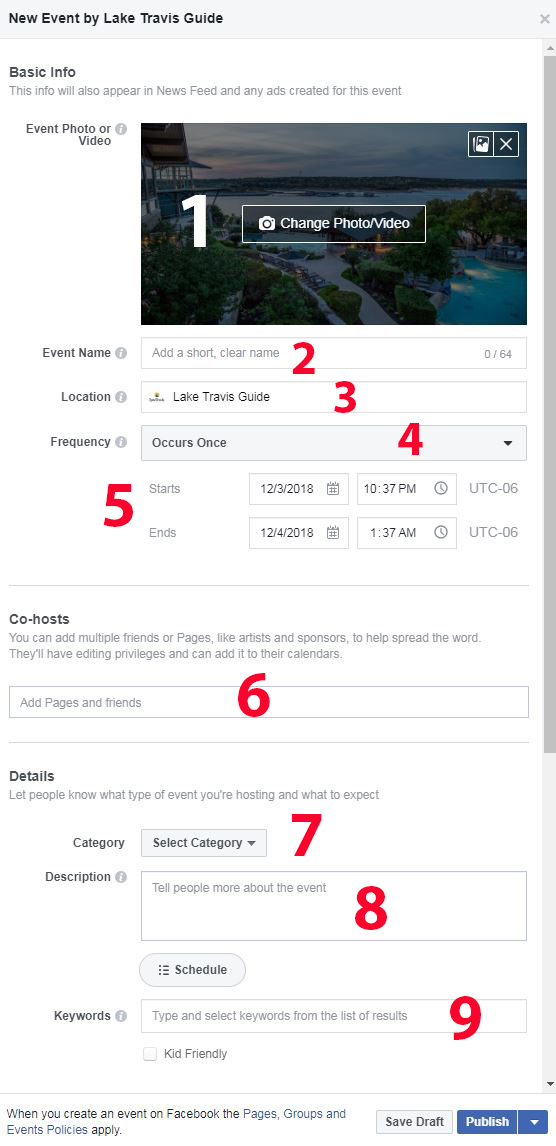The detailed image caption is as follows:

At the top of the image, there's a light gray header. Towards the left side of this header, in bold black lettering, it states "New Event by Lake Travis Guide." Beneath the header, there is a medium gray divider that forms the bottom border of the header. The background transitions into white, and on the left side in black lettering, it reads "Basic Info." Just below this, in small gray lettering, there's a note explaining, "This info will also appear in newsfeed and any ads created for this event." 

Further down on the left, in bold, small black lettering, it says "Event Photo or Video." To the right of this text at the top, there is a filled gray circle containing an italicized white eye icon in the middle. Adjacent to the circle, there’s a banner image that appears to be a photo of a resort surrounded by numerous trees and blue water, featuring visible people and waves. Within this banner, there is a large rectangular area with a white border that includes a white camera icon and the white text, "Change Photo/Video."

Below this banner, the content transitions into editable fields. The first field on the left is labeled "Event Name" with an eye icon next to it, and includes an input field for entering text. A small red number "2" overlays this section, marking it as the second step. The next field is labeled "Location," also accompanied by an eye icon and an input field. This section has a small red number "3" overlay, indicating it as the third step. 

Further down, the text "Frequency" is displayed in small black bold lettering, followed by the note "Occurs Once," and a dropdown menu indicated by a black arrowhead on the right. This section is marked with a small red number "4," designating it as the fourth step. Lastly, the fifth step section, labeled "Starts," includes fields for entering a start date and time, shown here as "12/3/2018 at 10:37 PM" as well as an end date and time, displayed as "12/4/2018 at 1:37 AM."